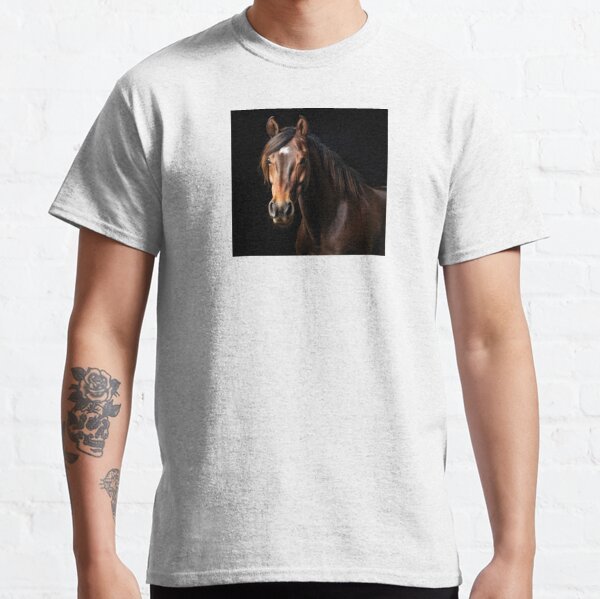This close-up photograph captures the torso of a tall male wearing an extra-large white t-shirt, prominently showcasing a square image of a chestnut horse set against a black background on the upper center of the shirt. The horse, with a white star on its forehead, flared nostrils, and a black mane swept to the left, is the main focus of the image. The man, who has a pale complexion, stands against a white painted brick wall, with his head cropped out of the frame. His arms are relaxed by his sides, revealing a tattoo of a skull with a rose on his right arm. The lower part of the photo hints at black denim jeans but is cut off at the waist. The photograph's emphasis appears to be on the t-shirt's design featuring the striking image of the horse.